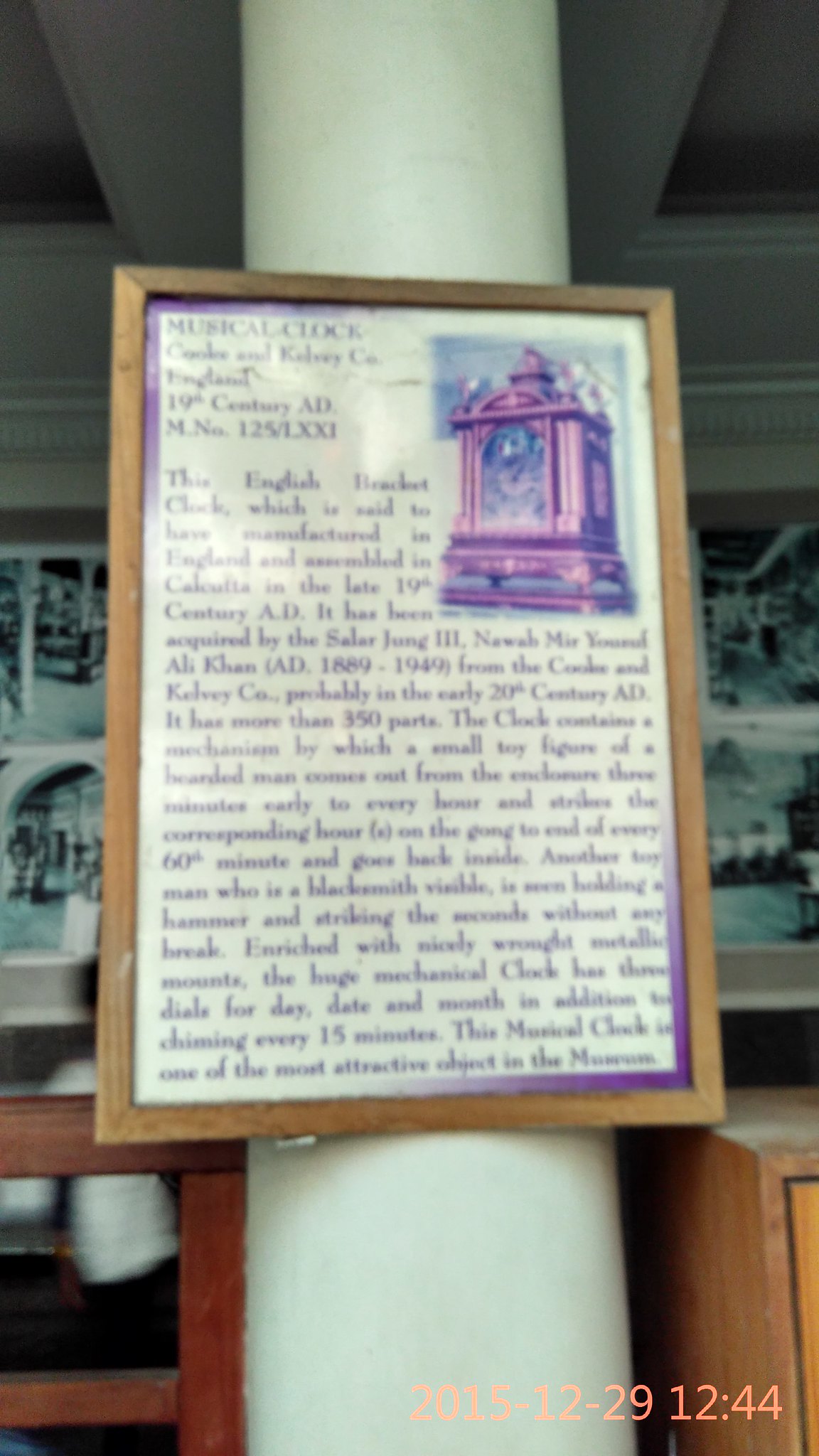In this vertically-oriented, rectangular image, a framed photograph is prominently displayed on a large white cylindrical pillar, seemingly within a museum or gallery space. The photograph is encased in a brown wooden frame and stands vertically against the pillar. The image itself features an English bracket clock, alongside detailed yet hard-to-read text in a decorative old English font. The clock, depicted with dials for day, date, and month, chimes every 15 minutes and traces back to the late 19th century, having been manufactured by the Cook and Kelvey Company of England and assembled in Kolkata, India. The text surrounding the clock provides historical context about its origins and significance.

At the lower right corner of the photograph, the timestamp "2015-12-29 12:44" is visible in a peach-colored font, indicating when the image was captured. In the background, the setting includes various artworks or photographs, predominantly in black and white, framed in light gray. Adjacent to the pillar, there is a rectangular wooden box or shelf and a low bookshelf or possibly the top of a ladder, made of brown wood, adding to the ambiance of the space. Overall, this detailed portrayal encapsulates the essence of the museum exhibit and the historical artifact it features.